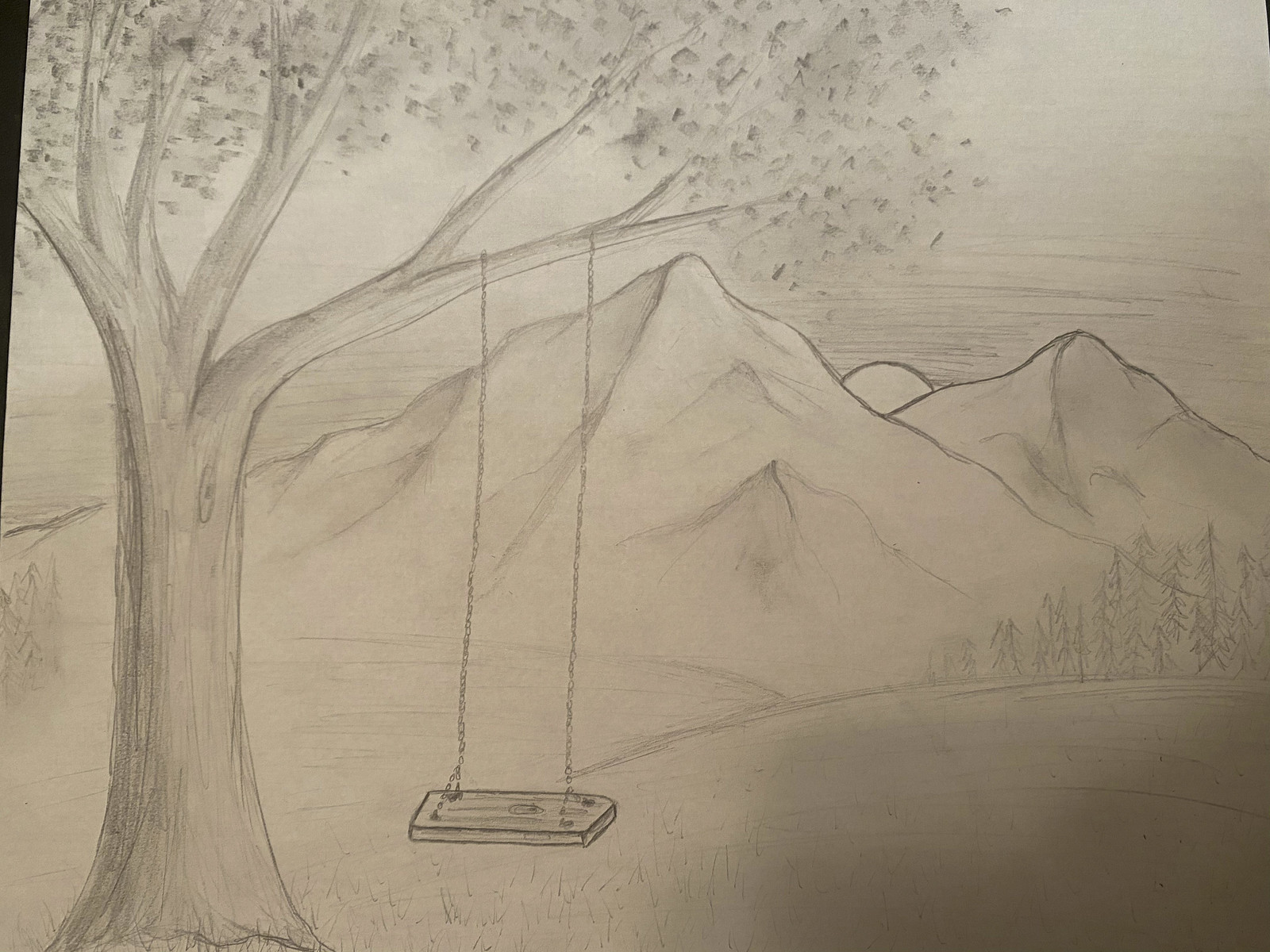This is a detailed pencil drawing rendered in black and white on standard white stock paper. The focal point of the artwork is a large tree in the foreground, adorned with a swing. The swing features a wooden base suspended by sturdy chain links. Behind the tree lies a serene meadow that stretches towards a range of mountains in the far background.

The setting sun, perfectly positioned between the two mountain peaks, casts a gentle light over the scene, suggesting either twilight or dawn. To the middle right of the mountains, a dense cluster of trees forms a small forest, while to the middle left, additional trees are faintly visible, adding depth to the composition. The overall scene captures a tranquil moment in nature, beautifully detailed with the artist's skillful use of shading and texture.